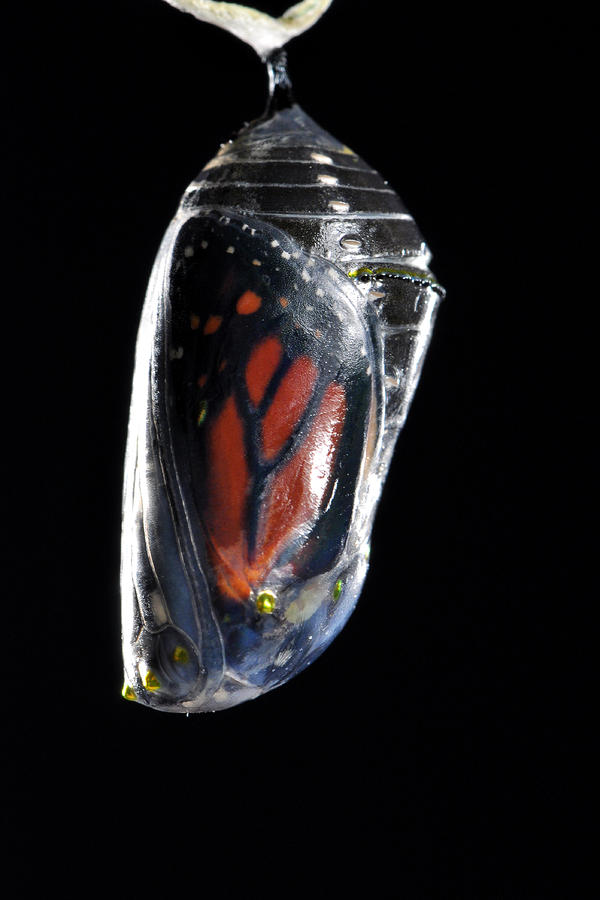The photograph, presented in portrait orientation, captures a detailed and striking image of a monarch butterfly in its chrysalis stage suspended from the top edge on a silken thread against a solid black background. The chrysalis, a transparent, oblong structure with a conical slope at the top, has an intricate, glass-like appearance. Inside, the delicate wings of the monarch butterfly are distinctly visible, featuring vibrant orange centers with intricate black veins running through them. Reflective lighting, which might be either natural or artificial, illuminates the chrysalis from both sides, creating bands of light that enhance the clarity and elegance of the scene.